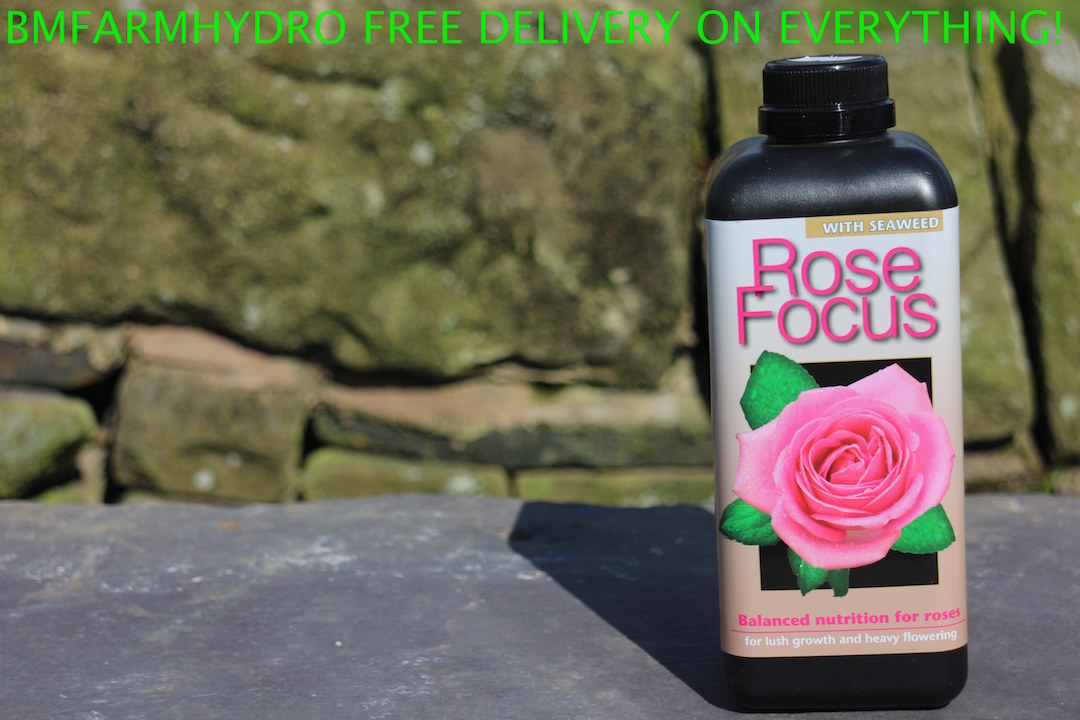In the foreground of this rectangular image, there is a black bottle with a black cap, prominently labeled "Rose Focus" in bright pink text. The label features a large pink rose with green leaves, and below the rose, it reads "Balanced Nutrition for Roses" in pink lettering, followed by "For Lush Growth and Heavy Flowering" in white text. At the top of the label, in small white capital letters on a pale yellow background, it states "With Seaweed." The bottle, positioned on a grey stone ledge that spans the width of the image, is part of a product advertisement likely intended for online or magazine use. In the background, there's a wall composed of various sized stones with earthy tones and traces of moss, providing a rustic backdrop. Above the bottle, in neon green capital letters, the text reads "BM FARM HYDRO - FREE DELIVERY ON EVERYTHING." Overall, the image effectively highlights the plant food product, emphasizing its benefits for roses with a natural, outdoor setting.